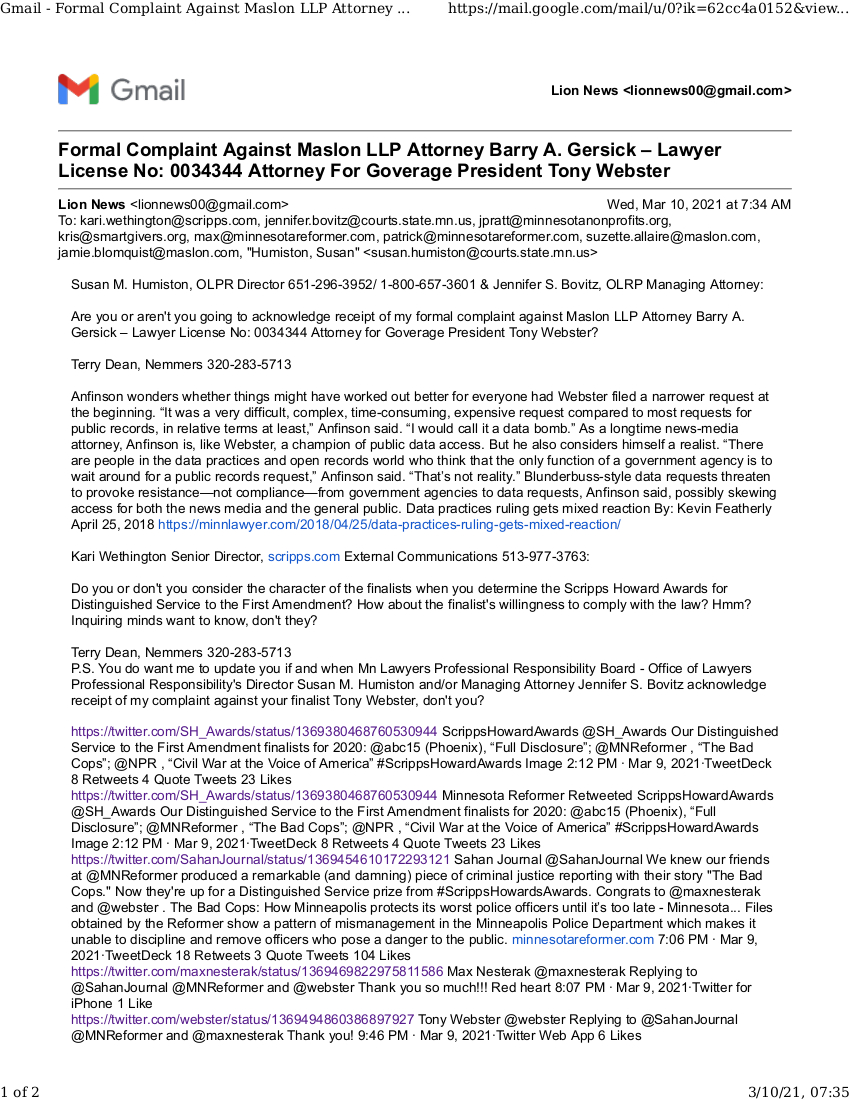In this image, a Gmail interface is displayed on a screen, featuring a formal complaint email against Mass Link LLP. On the top left corner, the Gmail and Google icons are visible. The subject line reads, "Formal Complaint Against Mass Link LLP R20," and includes a hyperlink, "Lion News," with the email address lionnews00@gmail.com.

The email is a formal complaint filed by Barry A. Jerzyk, a lawyer with license number 0034344, who represents Tony Webster, the President of Gove Ridge. The content below the heading of the email details the nature of the complaint. Various individuals are copied on the email: kari.within@scripps.com, jennifer.bovitz@course.state.mn.us, and jppratz@minnesotaprofits.org.

The colors in this image—featuring the Gmail logo and interface—are predominantly red, yellow, blue, and green, set against a white background with black text.